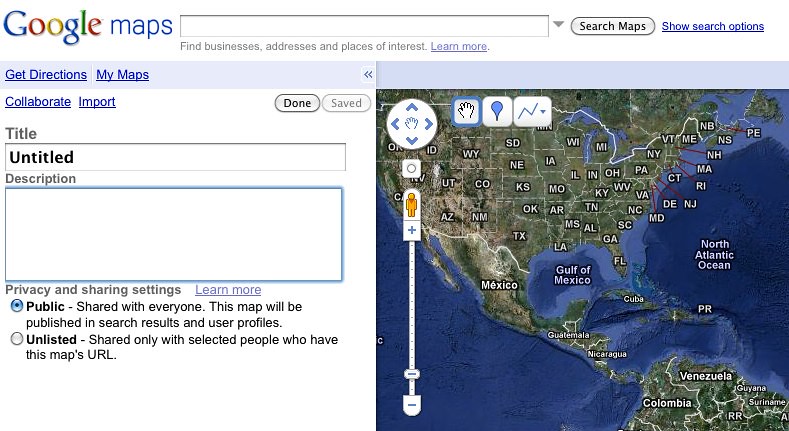The image appears to be a screenshot of an older version of Google Maps, likely from 10 to 20 years ago, depicting a user interface that is simpler and more rudimentary compared to modern interfaces. In the upper-left corner of the screen, the familiar multicolored "Google" logo is present, accompanied by the word "Maps" in blue. Below this, there is a search box where users can enter addresses. Directly under the search box, a line of text reads, "Find businesses, addresses, and places of interest." A "Learn more" hyperlink follows this text.

To the right of the search box, a down arrow is present along with a "Search Maps" button and another hyperlink labeled "Show search options." 

The displayed map provides a broad view encompassing most of the continental United States, parts of Latin America, the Caribbean, sections of northern South America, the North Atlantic Ocean, the Gulf of Mexico, and parts of the Pacific Ocean.

On the left side of the screen, there are several hyperlinks for different functions, such as "Get directions," "My maps," "Collaborate," and "Import." Below these, a small textbox labeled "Title" appears to be empty, alongside a larger textbox under the header "Description," which is also devoid of content.

Towards the bottom of the screen, there is a section labeled "Privacy and sharing settings." The public sharing option, which allows the map to be published in search results and visible on user profiles, is currently selected. An unselected radio button beneath this option is labeled "Unlisted," indicating that the map would only be shared with people who have the map's URL if this option were chosen.